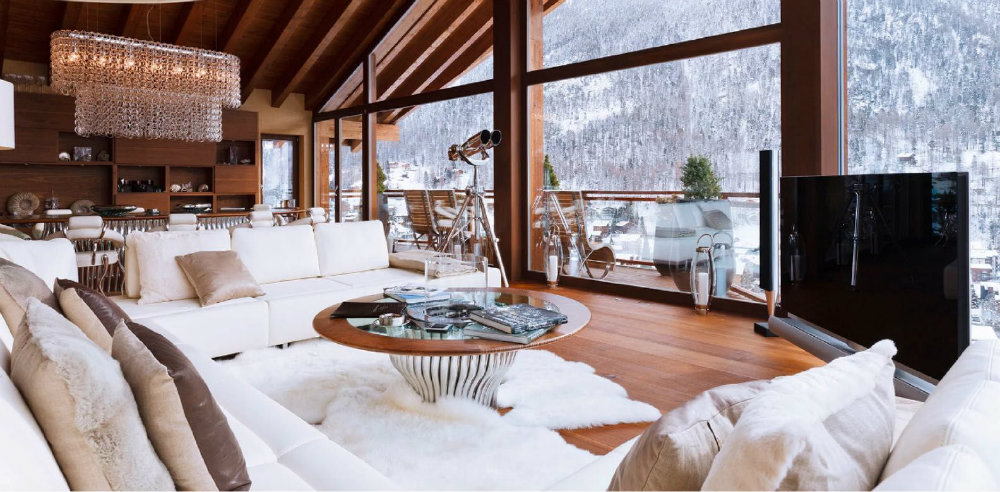The image depicts a luxurious and opulent living room in a wooden mountain home, possibly located in the snowy regions of the Alps or Colorado. The warm living space features extensive use of wood, with wooden floors, walls, and ceilings, creating a cozy and inviting ambiance. Dominating the room is a large horseshoe-shaped white couch adorned with numerous pillows, sitting atop an ultra-soft white rug. A round glass and wooden coffee table is positioned in front of the couch.

The room boasts floor-to-ceiling, see-through plate-glass windows that offer breathtaking views of a majestic snow-covered mountain and snow-laden trees. A pair of golden binoculars on a tripod stands ready for a closer inspection of the stunning scenery. 

A massive glass jeweled chandelier hangs from the cathedral ceiling, illuminating a large dining table positioned at the back of the room. Modern comforts are not overlooked, with a large big-screen TV and speakers strategically placed for an optimal viewing experience. The overall atmosphere combines rustic elegance with contemporary luxury, making it a perfect winter retreat.